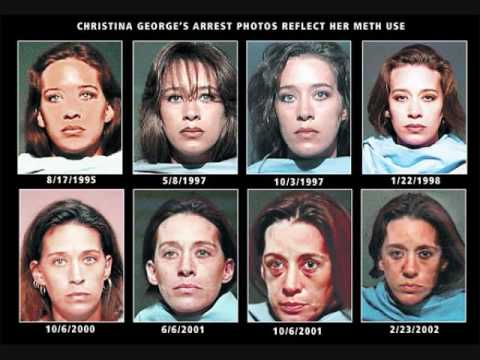This image is a collage of eight arrest photos of Christina George, documenting her downward spiral from meth use over seven years. The background is black, with a caption in white font at the top reading: "Christina George's arrest photos reflect her meth use." The images are arranged in two rows of four.

In the first photo dated 8-17-1995, Christina appears relatively healthy with light skin and shoulder-length dark brown hair, some reddish highlights, and a neutral expression. The second photo, dated 5-8-1997, shows her with similar appearance but with wispy front bangs.

By the third photo dated 10-3-1997, she looks slightly thinner, her hair darker and wavy, flopping to one side. The fourth photo, dated 1-22-1998, shows her with reddish highlights again and half-closed eyes, but a similar hairstyle to her initial photo.

In the second row, the photo dated 10-6-2000 reveals a noticeable deterioration with very dark hair at the top and lighter at the ends, hoop earrings, and a significantly thinner face. The sixth image from 6-6-2001 shows her even more gaunt, with short, unkempt hair and possible bruising on her forehead.

By 10-6-2001, Christina looks severely unhealthy, with red bags around her eyes and sores on her face, her weight markedly reduced. The final photo, dated 2-23-2002, depicts her nearly unrecognizable with very short hair, scabs covering her face, and a shell of her former self.